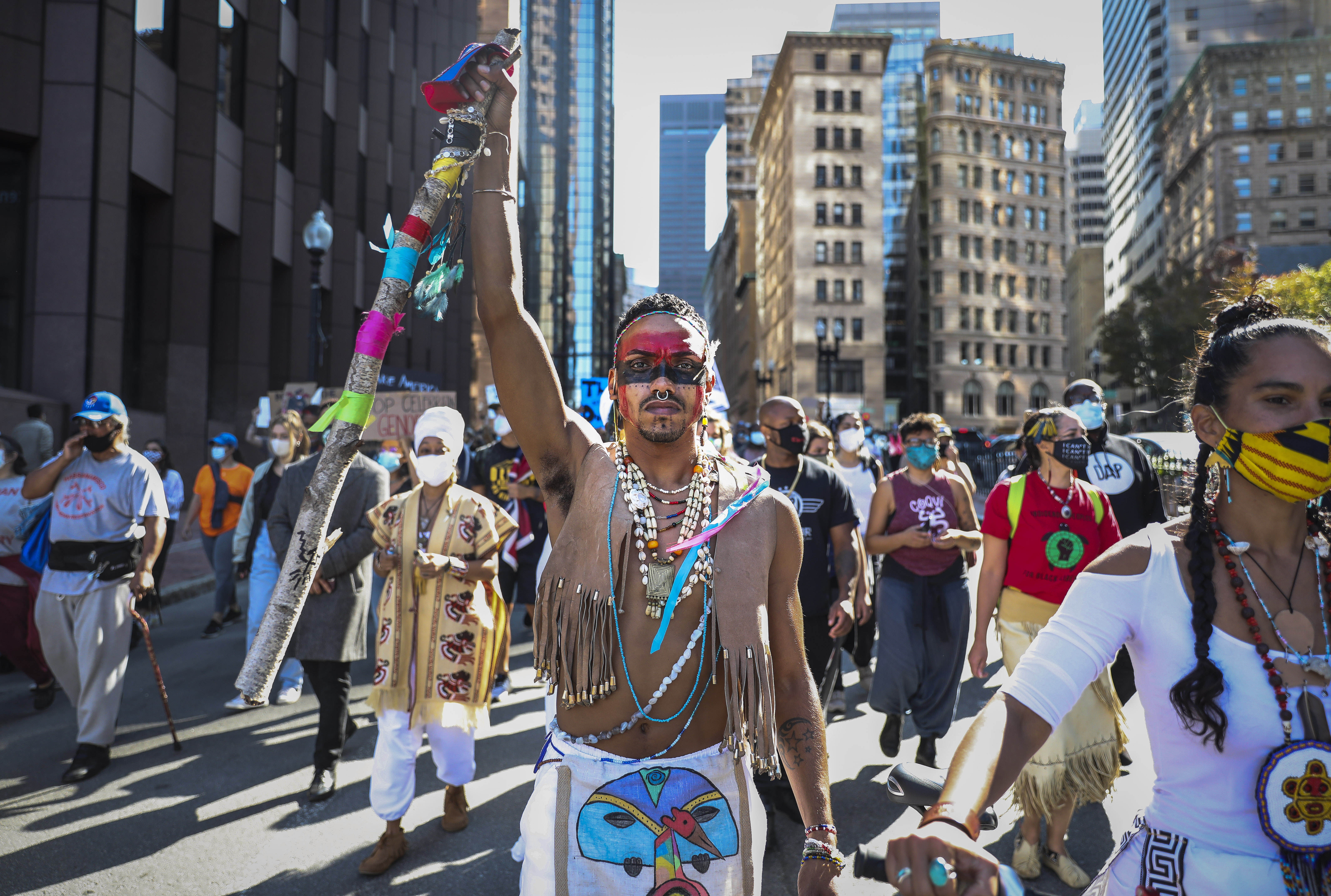The photograph captures a vibrant event on a bustling street, likely in New York City, featuring what appears to be a Native American parade or protest. Central to the image is a man dressed in traditional Native American attire, standing directly in the middle of the frame. He has red and black paint around his forehead and eyes, a nose ring, and wears a tan suede vest with fringe ending in brass details. Around his neck, he sports white shells, and he holds aloft a colorful stick adorned with black, yellow, red, blue, purple, and yellow. The man looks directly into the camera and is dressed in an outfit resembling a man’s dress, which features a drawing of a mushroom. Beside him, a woman similarly dressed in Native American-style clothing and wearing a necklace of beads walks along. Behind them, other individuals, also in traditional costumes, are visible, all framed by tall buildings that encircle the scene from left to right. The event, filled with bright pinks, lime green, blue, red, yellow, black, brown, tan, beige, and orange, seems to be a celebration or a protest, rich in cultural expression and activity.